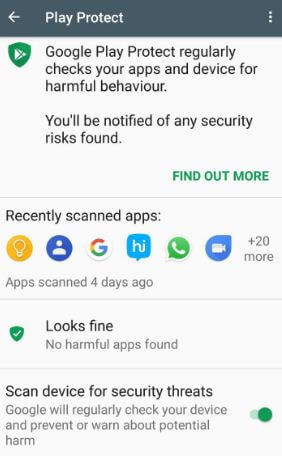A screenshot captures a section of the Google Play Store app on an Android phone, specifically the "Play Protect" feature. The header reads, "Google Play Protect regularly checks your apps and device for harmful behavior. You'll be notified of any security risks found." There's a link to "Find out more" about this feature. 

The middle section, titled "Recently scanned apps," showcases a list of app icons such as Google Keep, Contacts, and Assistant, indicating active protection against malicious activity. Each app was scanned four days ago.

Following this, the screen assures the user that no threats were detected with a message, “It looks fine,” accompanied by a green shield icon with a check mark.

At the bottom, there's a toggle switch labeled "Scan device for security threats," which is currently turned on. The description below it states, "Google regularly checks your device and prevents or warns about potential harm," highlighting the continuous protection provided by Play Protect. This ensures that the user's device is shielded from malicious apps, making the Google Play Store a logical placement for such security measures.